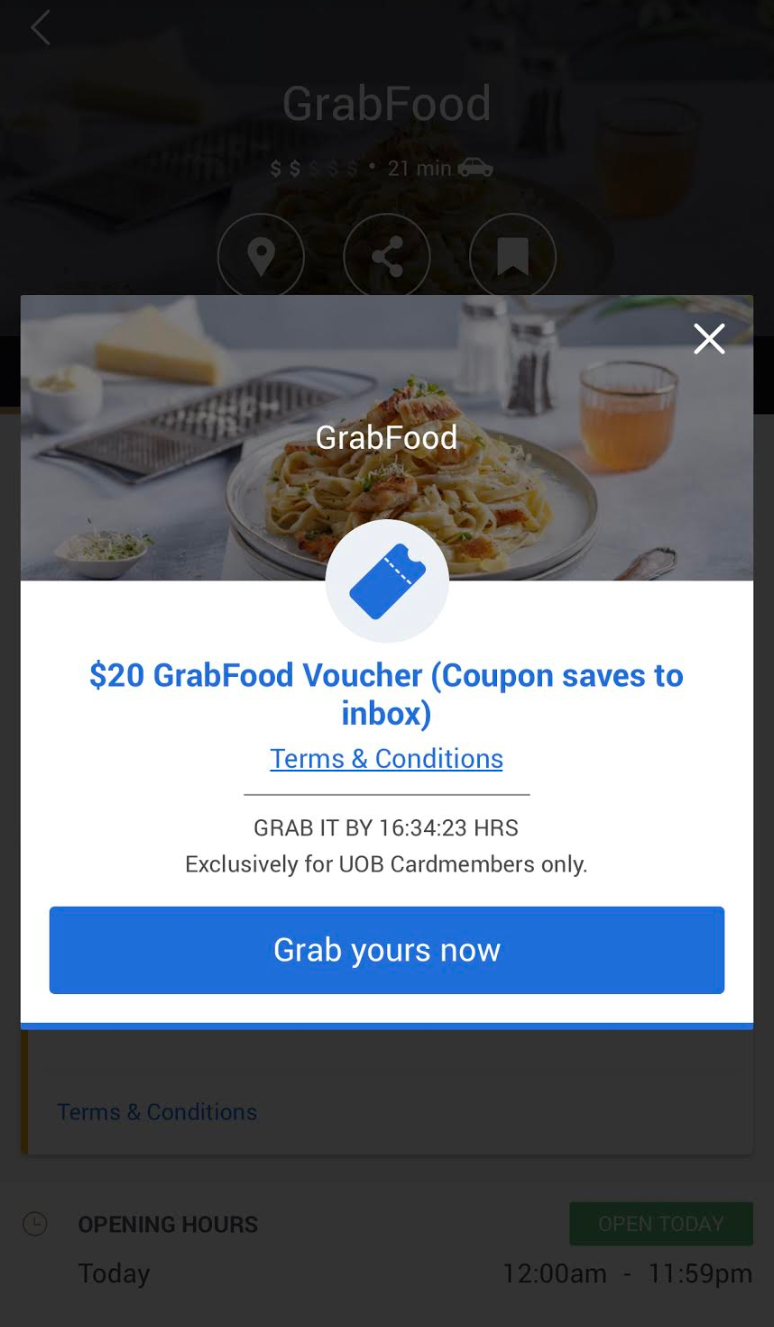This image depicts the user interface of a GrabFood application. The background of the interface is a grayed-out black, indicating the presence of an active pop-up window. At the top of the grayed-out background, "Grab Food" is displayed in white font accompanied by a rating of two dollar signs out of five, which likely represents the cost level. The information "21 minutes by car" is also visible, providing an estimated delivery time.

The interface includes three circular icons placed side by side: an address pin icon, a share icon, and a bookmark icon, all situated above an image of a table with a plate of food.

The central focus of the pop-up window reiterates "Grab Food" and prominently displays the same table and plate of food image. Below this image is a circular element that extends into the lower section of the pop-up window and contains a message stating "$20 Grab Food Voucher Coupon saved to inbox." To the right of this message is a conspicuous blue button with the label "Grab yours now."